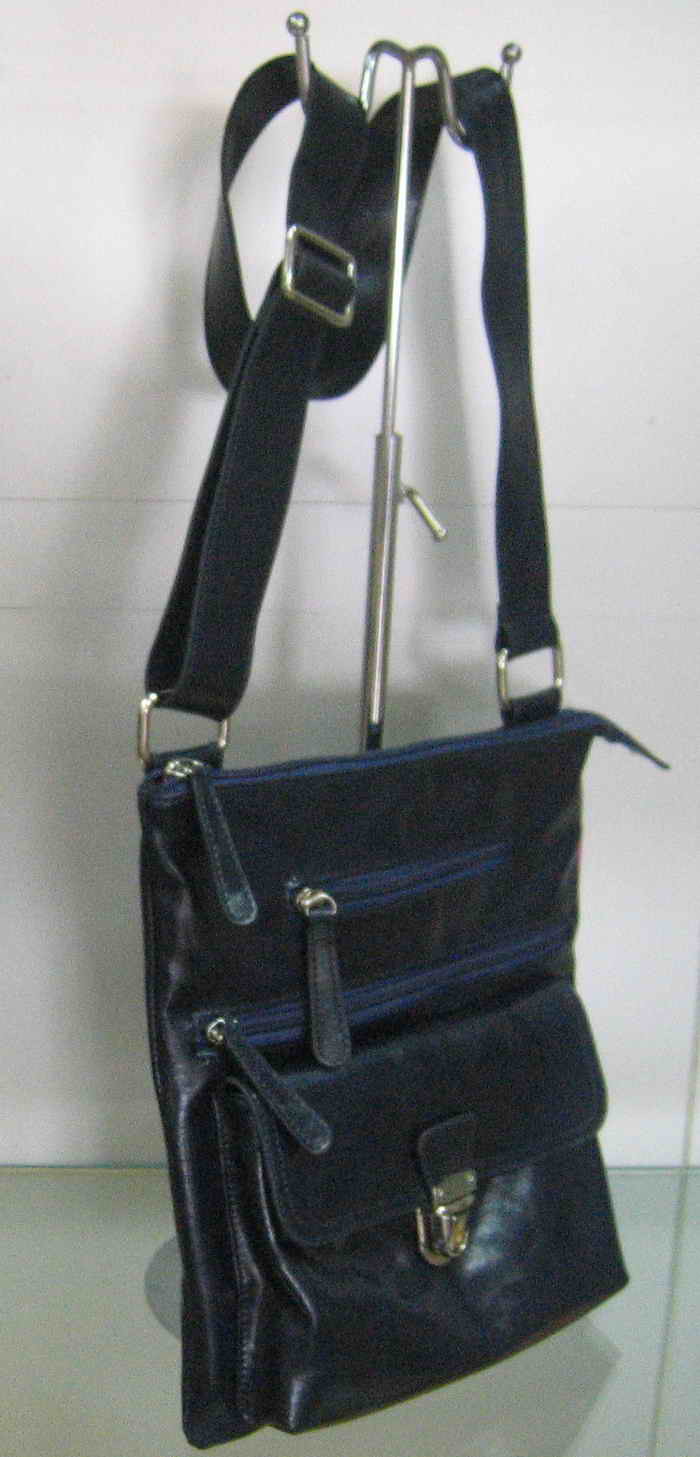This image features a sleek and slim crossbody bag or purse, which is suspended from a silver metal hanger. The bag, made of shiny leather, has a dark hue that alternates between black and deep navy depending on the light. It is equipped with multiple storage compartments, including three zippers with long pulls and an additional pouch with a clasp for secure closure. The bag hangs by a long strap that suggests it can be worn over the shoulder. Behind the bag is a white wall, and the lower part of the image shows a greenish tabletop surface, with no other items present in the scene.